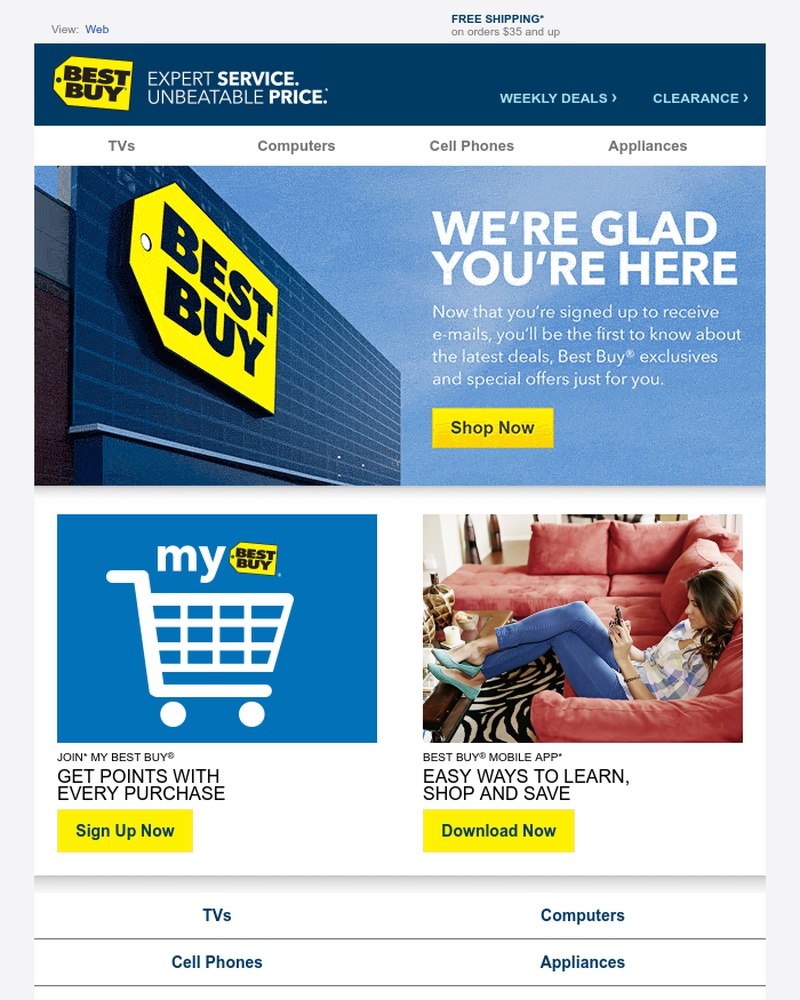**Detailed Caption:**

This image is a detailed screenshot from the Best Buy website, likely viewed on a tablet given the layout. The page features a dark blue header bar with the Best Buy logo prominently displayed in the upper left corner. The logo consists of black text with a distinctive yellow tag. Next to the logo, the slogan "Expert Service, Unbeatable Price" is displayed, with "Service" and "Price" in bold for emphasis. To the right, the navigation options include "Weekly Deals" and "Clearance."

Beneath the header, a white strip contains the main navigation menu with categories such as TVs, Computers, Cell Phones, and Appliances. The central part of the screenshot features a large hero image of a Best Buy store exterior, showcasing the recognizable blue tiled façade and a 3D store sign. The left of the image shows brown bricks or cinder blocks, adding texture to the building's appearance. 

Superimposed on the hero image is a welcoming message: "We're glad you're here. Now that you signed up to receive emails, you'll be the first to know about the latest deals, Best Buy exclusives, and special offers just for you." Below this message is a prominent yellow "Shop Now" button, inviting users to explore current promotions.

The lower section of the screenshot is divided into two parts. On the left, there's an advertisement for the "My Best Buy" membership program, which offers points with every purchase and a sign-up invitation. On the right, an image depicts a woman lounging on a pinkish-red sectional couch with her feet up, browsing a smartphone. This section promotes the Best Buy mobile app with a tagline that highlights its convenience: "Easy ways to learn, shop, and save. Download now."

Finally, at the bottom of the screenshot, the navigation categories are reiterated in blue text: TVs, Computers, Cell Phones, and Appliances, making it easy for users to navigate to their desired products.